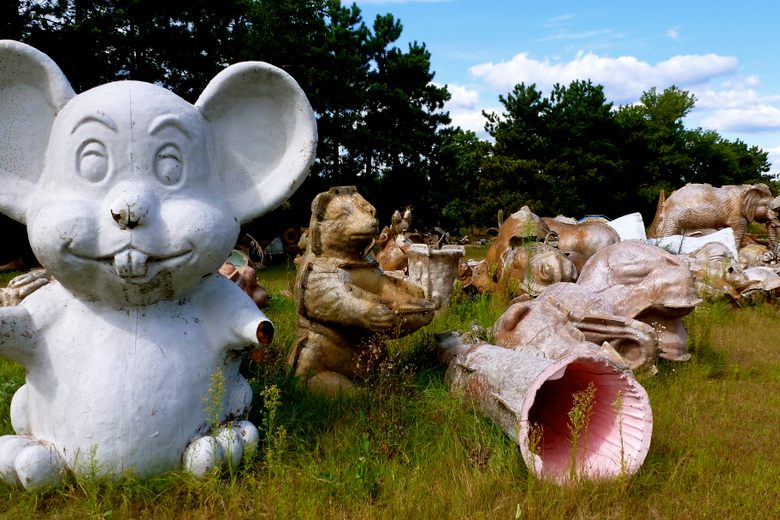In this photograph taken outdoors during the day, we see a collection of garden statues set against a backdrop of lush grass. Dominating the left side of the composition is a large, cartoon-style mouse statue, crafted from white cement. This figure, sitting comfortably and appearing to be about four or five feet tall, shows wear with its left paw visibly missing, presumably broken off. The mouse sports a cheerful smile with two prominent buck teeth, large ears, partially lidded eyes, and defined eyebrows, lending it a whimsical expression.

Adjacent to the mouse statue to the right is a bear statue, seemingly designed to hold a bowl, which likely serves as a birdbath. This bear figure adds a functional element to the garden display. Other statues are clustered together further right, but their exact forms are difficult to distinguish amidst the ensemble. They collectively present a mix of various brown tones and hints of light salmon pink, creating a diverse yet harmonious assembly of outdoor art.